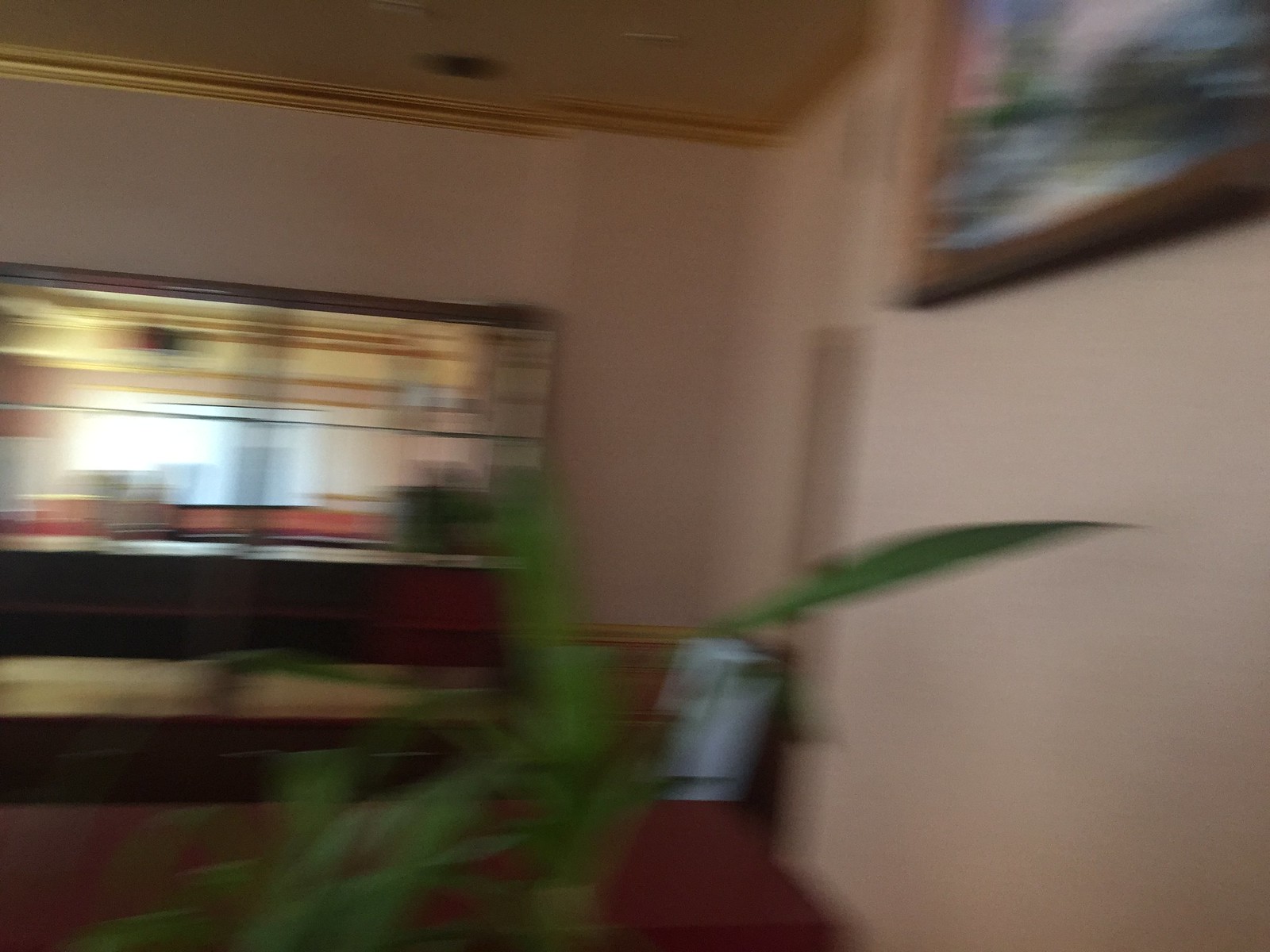This image is a slightly wider-than-tall, blurry photograph taken indoors, possibly in a hotel lobby or bedroom, characterized by a distinct hotel aesthetic. The photo appears to have been captured while the camera was moving rapidly from left to right. In the foreground, partially obstructing the view, are the long green leaves of a potted plant situated near a wall. The room features very plain walls, accented by gold crown molding where the walls meet the ceiling. A red or dark reddish-brown carpet covers the floor.

In the background, against the far wall, there is a reflective surface, possibly a mirror or a TV with a significant glare. The right wall hosts a large rectangular painting that looks like a landscape, though it's cut off slightly due to the focus on the corner between the right wall and the far wall. Light enters the room from windows directly ahead, offering a glimpse into another room, but the details remain obscure due to the blur. Additionally, there is a closed door on the right wall and a bench-like piece of furniture possibly located under the window. Ceiling lights are visible, contributing to the room's illumination.